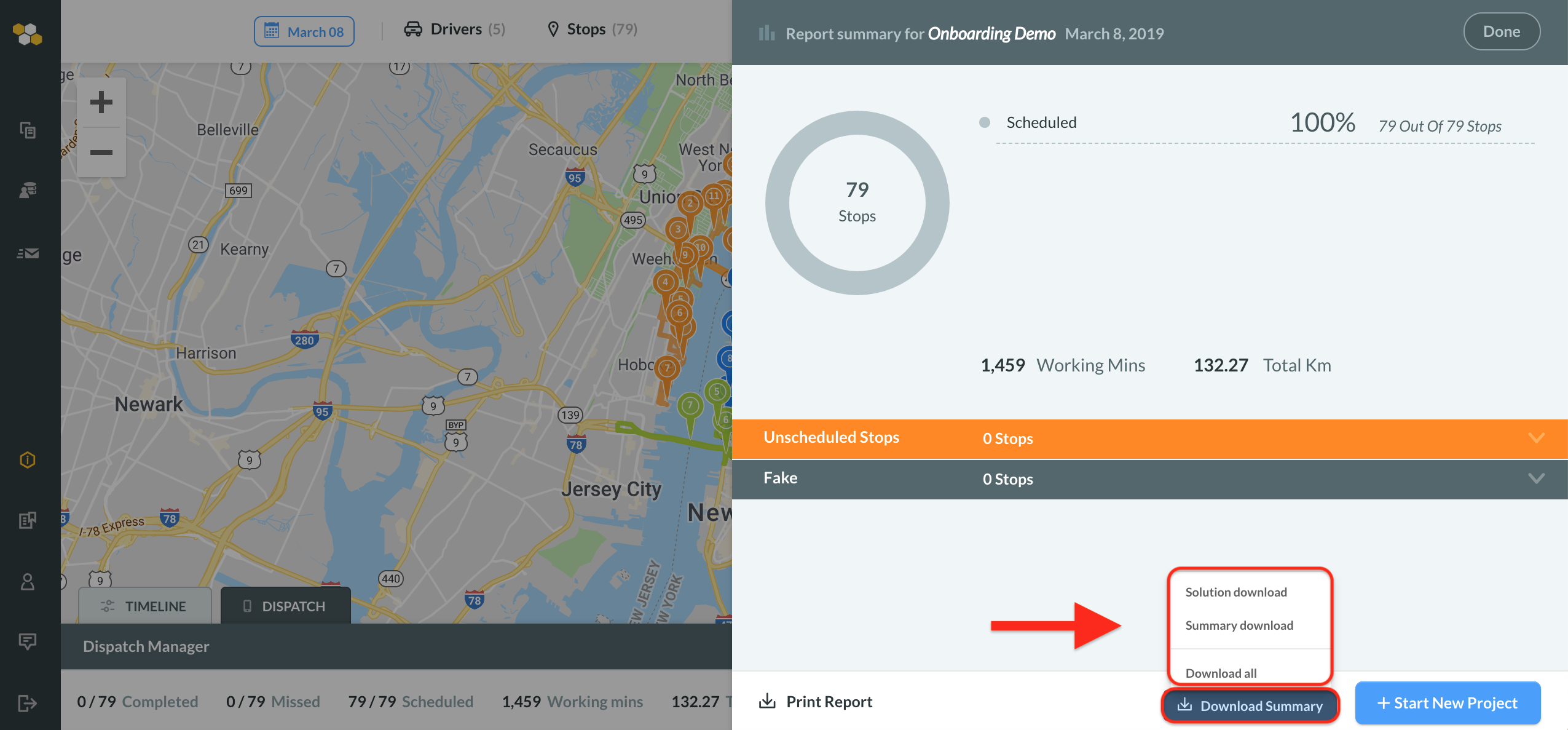Detailed Caption: 

The image is a composite of two distinct sections. On the left side, there is a map of the Newark, New Jersey area, featuring a range of geographical and infrastructural details. The map is slightly tinted darker for clarity, showcasing highways in yellow, bodies of water in blue, and various town names, including Newark, Jersey City, and other smaller towns. This section also includes a black sidebar with menu buttons and a label at the top that likely reads "Drivers and Streets." Additionally, a black toolbar at the bottom contains various terms and numbers, presumably related to the map's data or controls, with a label possibly indicating a management function.

On the right side of the image, a report summary is displayed. The report is titled "Report Summary for Custom" with some illegible text due to the small print. The report date is noted as March 8, 2019, with the term "Done" marked next to it. Below this, the number 79 is encircled, indicating a task completion status, followed by the words "Scheduled 100%" and "79 out of 79." Further down, additional statistics are presented: "1,454 Working," "132," and "27," possibly denoting work-related metrics. These figures are accompanied by an orange and gray bar graph.

At the bottom right, a red arrow points to the right, accompanied by text in a red box, suggesting further instructions or important information. Additionally, two blue buttons labeled "Download" and "Start Report" appear at the lower section, likely providing interactive options for the user.